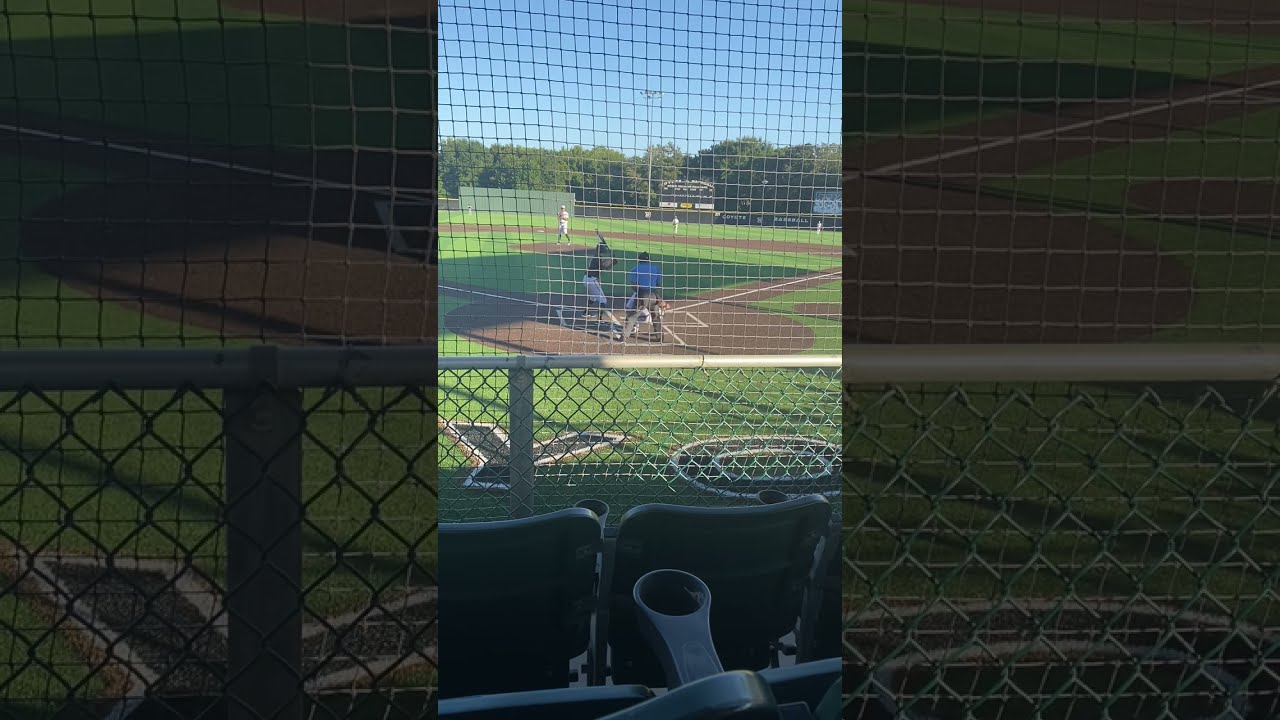This image captures a vibrant baseball game from a perspective behind home plate, viewed through the protective netting and a chain-link fence that slightly obscures the field. Central to the photo is a batter, noticeably attired in white pants and a dark-colored (possibly black) shirt, preparing to swing while an umpire—wearing a blue or possibly gray shirt—stands directly behind him. The catcher, barely visible, squats in position behind the umpire. Further visible details include the pitcher on the mound, dressed in an all-white uniform, and outfielders similarly clad in white, positioned in the distance.

The baseball field features a well-maintained green turf with the dirt diamond clearly marked in brown with white baselines. The stadium seats, some equipped with cup holders, appear in the foreground, likely suggesting the player's dugout area.

Beyond the field, various elements of the stadium can be seen: a green wall, a scoreboard displaying indistinct lettering (potentially reading "YO"), and lush trees surrounding the area. In the far distance, a light pole stands tall against a backdrop of buildings and a vivid blue, cloudless sky, encapsulating the sunny day's ambiance.